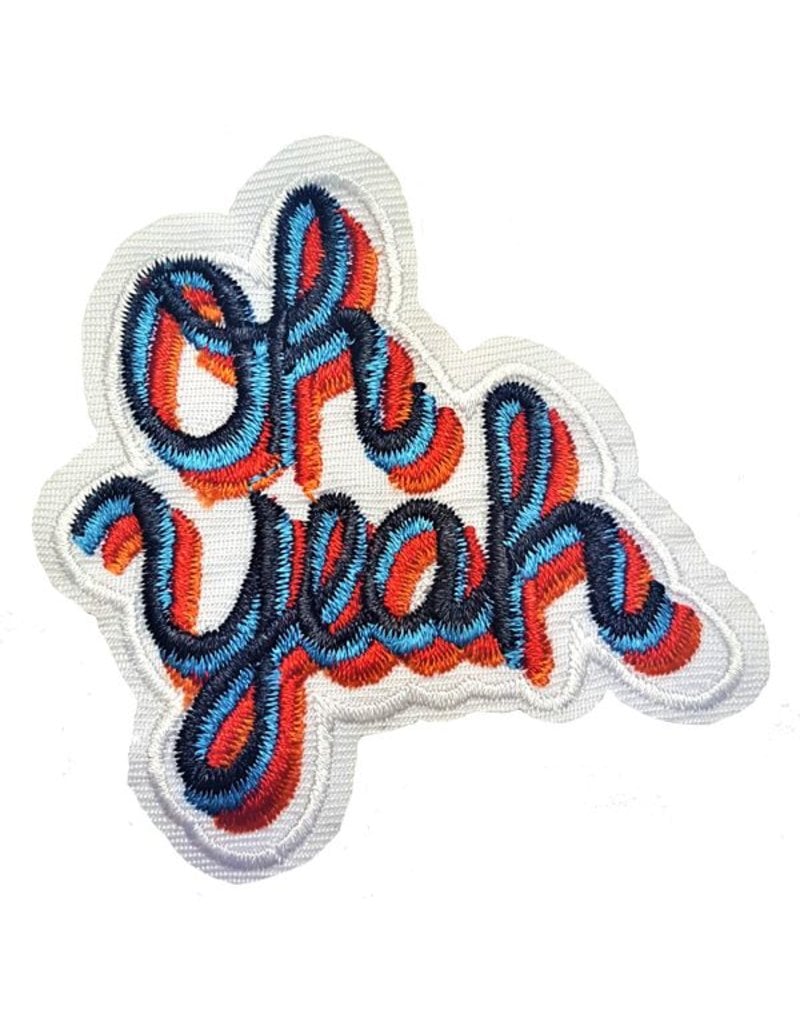The image showcases a detailed patch against a white background. The patch features the words "oh yeah" in a stacked, cursive font, with "oh" on the top line and "yeah" directly beneath it. The letters have a three-dimensional effect with layers of multiple colors: the uppermost layer is a dark navy blue, followed by teal, then red, and lastly orange. This layering gives the impression of light shining from the upper left, creating a dynamic shadow effect. The patch is outlined by a curvy white embroidered border that tightly follows the shape of the letters. Additionally, the entire patch, including its background and border, is seamlessly part of a larger piece of white fabric, enhancing the overall cohesive look.